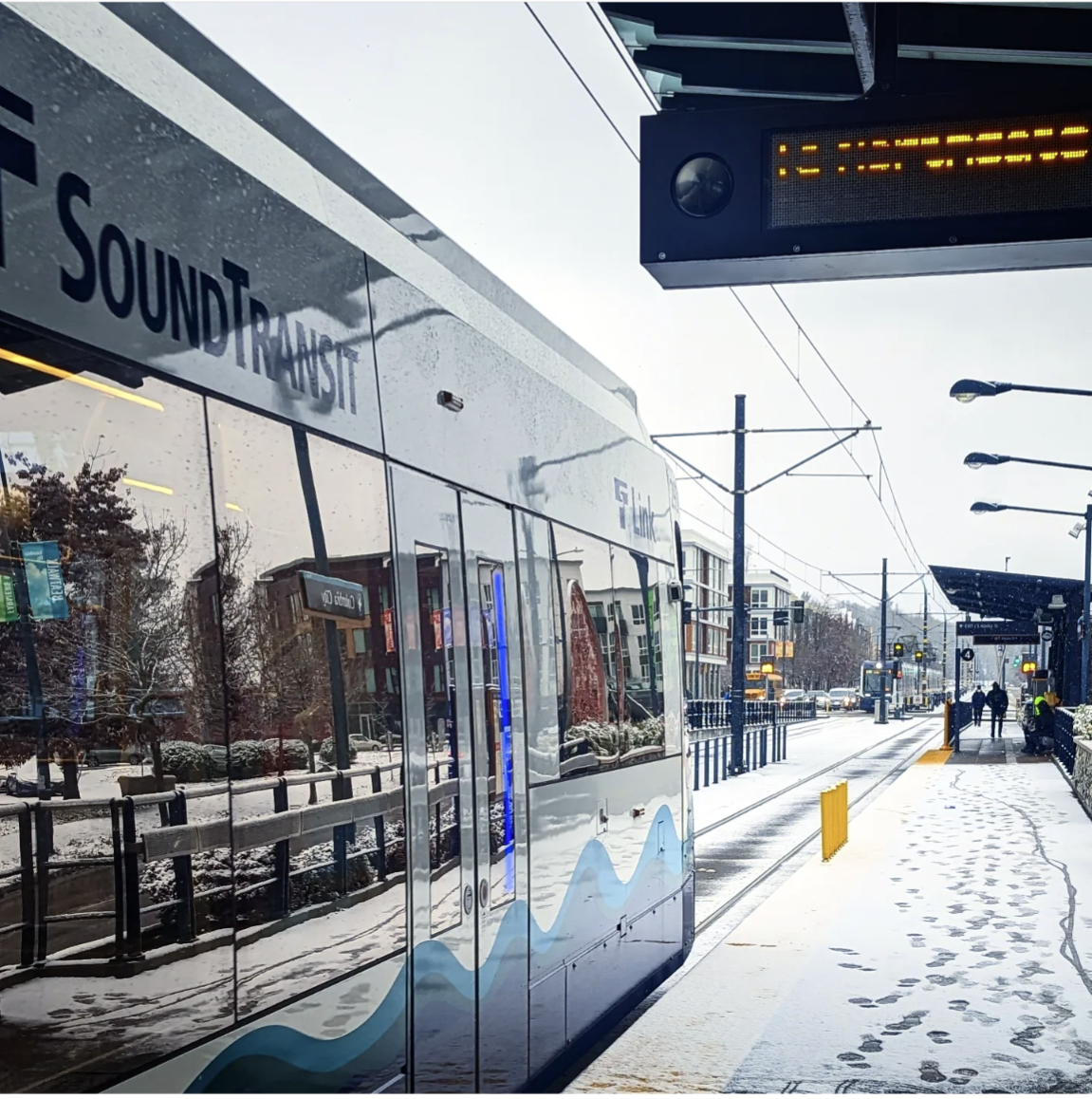The image captures a snowy, outdoor winter city scene with the focal point being a Sound Transit train entering a station. The rectangular photograph is slightly taller than it is wide, highlighting the train's shiny metal sides and large, tinted windows that mirror the surrounding urban landscape. The train features a blue wave pattern painted along its bottom, contrasting with its gray top. In the background, you can see city buildings, power lines, and street lights extending overhead. The ground is blanketed with snow, marked by numerous footsteps, and a snow-covered sidewalk runs alongside the train tracks. Down the sidewalk, under an awning shielding a patch from the snow, several people are visible in the distance. The reflective windows of the train capture the essence of the bustling city, while cars, traffic, trees, and distant hills are faintly visible, framing the vibrant urban scene.